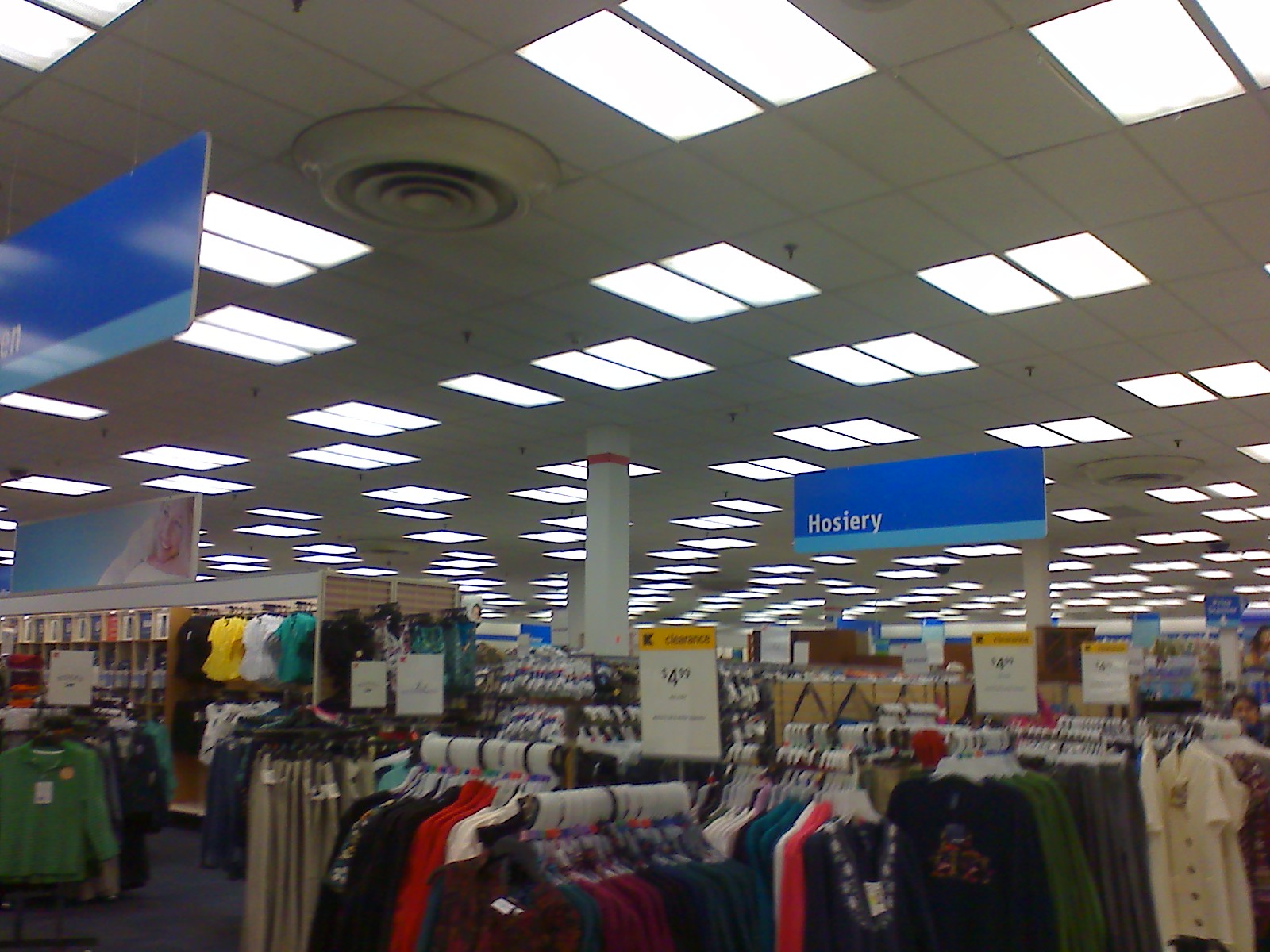This image captures the interior of a department store, characterized by its cool color scheme of blue and white with some grayish-red accents. The ceiling is white, adorned with rectangular, bright white lights and an overhead speaker. Hanging from the ceiling are large, rectangular blue-and-white signs indicating different sections, such as hosiery. The floor appears to be covered in gray carpet.

In the foreground, various racks display a multitude of multicolored shirts, neither particularly feminine nor masculine, along with a section containing long-sleeve shirts in red, black, and white priced at $4.99. Another nearby rack features khaki-colored long pants, and shorts can be seen on the left side. Also visible are sweatshirts in blue and green, some with designs on the front. The signs are clear and orderly, enhancing the organized layout of this corner of the store. There's even a beige and white rectangular price tag prominently displaying "$4.99." Overall, the store appears neat and meticulously categorized, creating an inviting shopping environment.